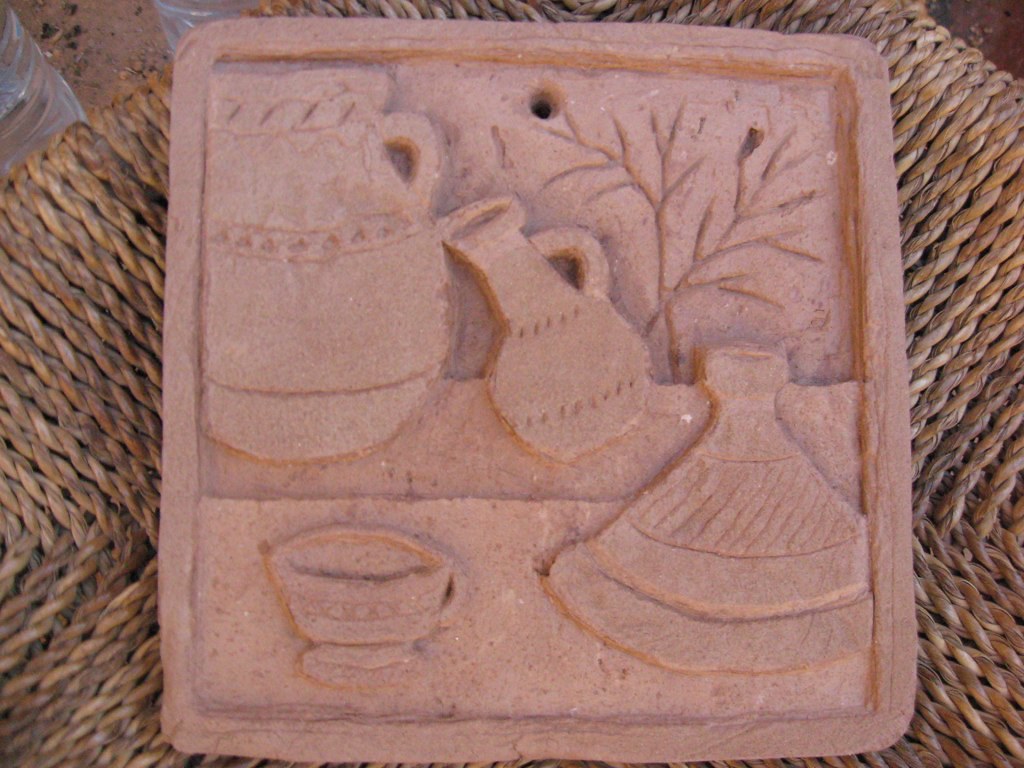This image showcases a detailed clay art piece that resembles a small ceramic tile, intricately decorated with a 3D effect despite its flat appearance. The artwork depicts an arrangement of various ancient kitchen items, prominently featuring several types of clay vessels, including a water jug, an alcohol flask, a large decorative vase with handles, and a small bowl or teacup situated in the bottom left corner. The central clay sculpture looks akin to an ancient kitchen table, enhancing the historical aesthetic of the piece. Additionally, there is a subtle etching of a tree in the background, adding depth to the design. The tile itself has a light brick red hue and rests on a tan-colored woven mat or stool. The photograph, likely taken indoors, captures the object from an overhead angle, emphasizing its intricate details and rustic charm. This clay art piece serves as a testament to traditional craftsmanship and evokes a sense of nostalgia, reminiscent of similar decorative items often found in kitchens.